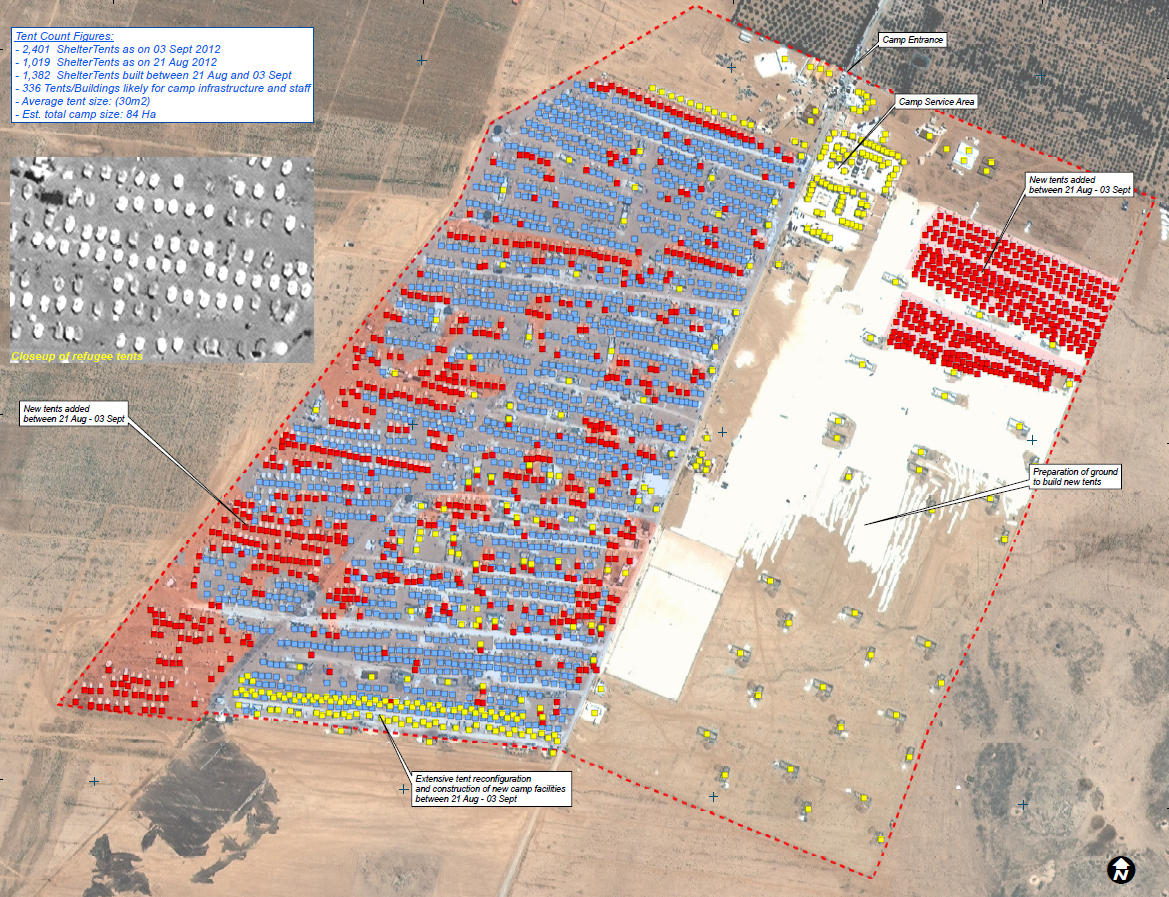The image is an overhead satellite view of an arid, desert-like region, characterized by a predominantly brown ground with minimal vegetation. At the top right of the image, numerous black spots are visible, though their nature is unclear. In the center, a triangular area features various colored markings—primarily red, blue, and yellow—alongside a road running through the middle. On the left side of this triangular section, multiple brightly colored areas can be seen. Adjacent to this area is a rectangular section marked by a prominent white spot with numerous red dots. Scattered around the map are white blocks with black text, some of which identify specific locations, such as "camp entrance" and "camp service area." In the top left, blue text on a white block is partially readable, mentioning "tent" and "tent count forces." Additionally, the image includes another smaller, black and white photo below the main map, offering a distant close-up of refugee tents. The map is framed with a dotted red line, further delineating the colorful regions within.